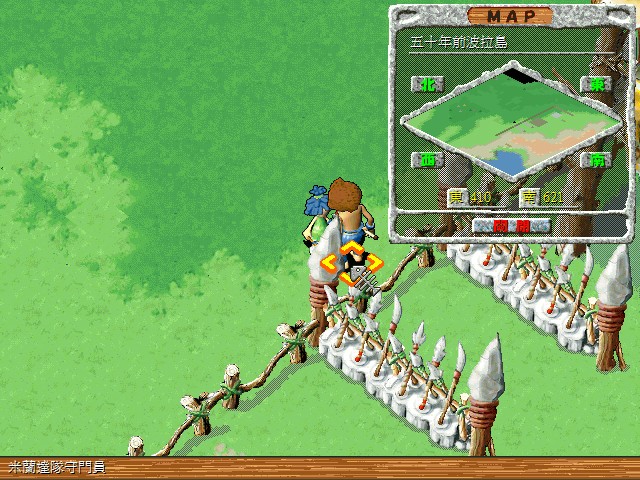The image depicts a scene from a video game, potentially designed for computers or mobile devices, with graphics reminiscent of early 2000s games. The interface is in Japanese or Chinese, as indicated by the text in the bottom-left corner. The scene features a light brown wood background with darker brown grains, stretching across the bottom. The grass in the foreground is displayed in two shades of green; the lighter green starts at the bottom and moves up the left side, gradually transitioning into a darker green, which has flecks of the lighter shade interspersed within it.

In the bottom right corner, there is a character with bushy brown hair, a brown body, and blue pants, though its specific nature is unclear. The character is positioned in front of what appears to be a base setup, which includes a brown fence running diagonally from the bottom left to the top right. In the top right corner of the image, a translucent map with a black outline is visible. The word "Map" is written in black on a brown background at the top of this in-game map.